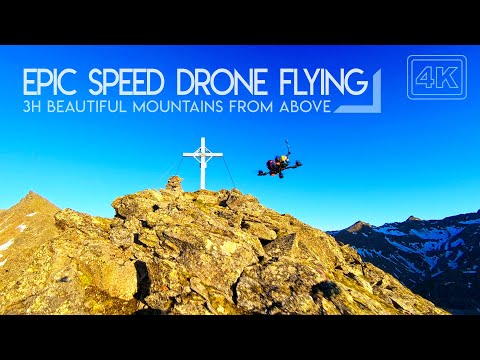A square, full-color image taken outdoors on a very sunny day depicts a dramatic aerial scene. The image is framed by thin black bars at the top and bottom, giving it a distinct, polished look. The sky transitions from a deep blue at the top to a lighter, glowing white closer to the horizon, emphasizing the bright natural light.

At the heart of the image, a light brown, rocky mountaintop stands prominently, adorned with a white cross at its peak. A sleek black drone, featuring yellow markings and distinctive circular elements, flies towards the cross, capturing an awe-inspiring scene. To the left of the mountaintop, a small patch of snow clings to a shaded area, adding contrast to the sunlit landscape.

In the background, snow-covered mountains stretch away into the distance, their peaks shrouded in shadows. The upper left corner of the image includes bold, white text reading, "EPIC SPEED DRONE FLYING," followed by "3H BEAUTIFUL MOUNTAINS FROM ABOVE" in a smaller font. The upper right corner features an outlined "4K" logo, indicating the high-resolution quality of the visual.

Overall, the image feels like a high-quality thumbnail or screenshot from a video, brilliantly showcasing the breathtaking beauty of mountainous terrain from above.